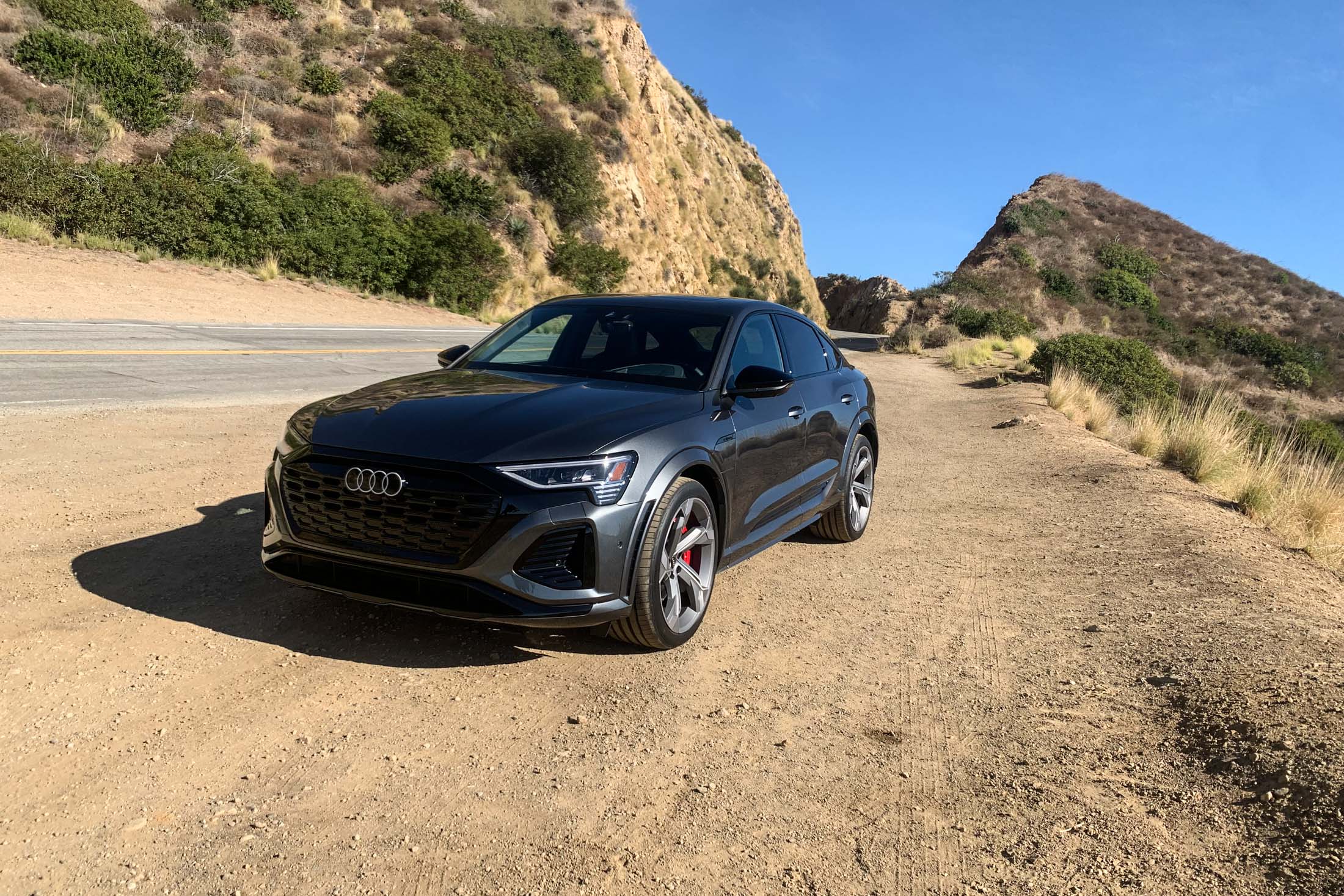The image captures a professionally shot photograph, potentially taken with a high-end consumer camera, of a sleek, black Audi sedan parked on a dirt shoulder beside a two-lane road in a desolate, arid outdoor area. The terrain features a blend of dirty, rocky ground with sparse, green bushes and some dry, yellowish grasses. The scene is set against the backdrop of small, rugged mountains and steep, rocky hills, which are sparsely adorned with foliage. The car, viewed from the front-left angle, showcases the distinctive four interlocking circles of the Audi logo, gleaming under the clear, sunny blue sky. The area is marked by dusty, tan-colored soil, contributing to the overall desolate and arid ambiance.